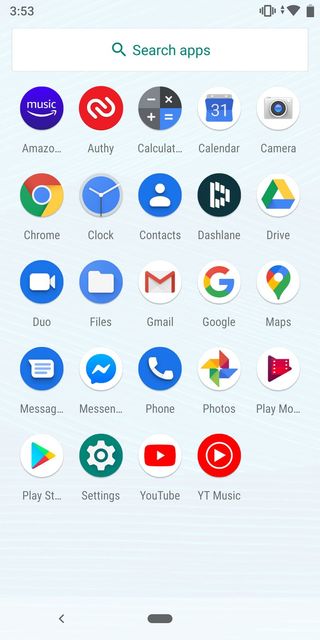The screenshot displays a smartphone's home screen. In the top left corner, there is a red status bar indicating a vibrating phone, Wi-Fi strength, and battery level. Below the status bar is a search apps bar. The screen features a grid of app icons, some of which are highlighted in blue. Notable apps include Music, Amazon, Calculator, Calendar, Camera, Chrome, Clock, Contacts, Dashlane, Google Drive, Gmail, Google Maps, Messaging, Messenger, Phone, Photos, Google Play Store, Settings, and YouTube. Also visible is YouTube Music. The background wallpaper depicts a scenic view of Hawaii. The bottom navigation bar has a left arrow.